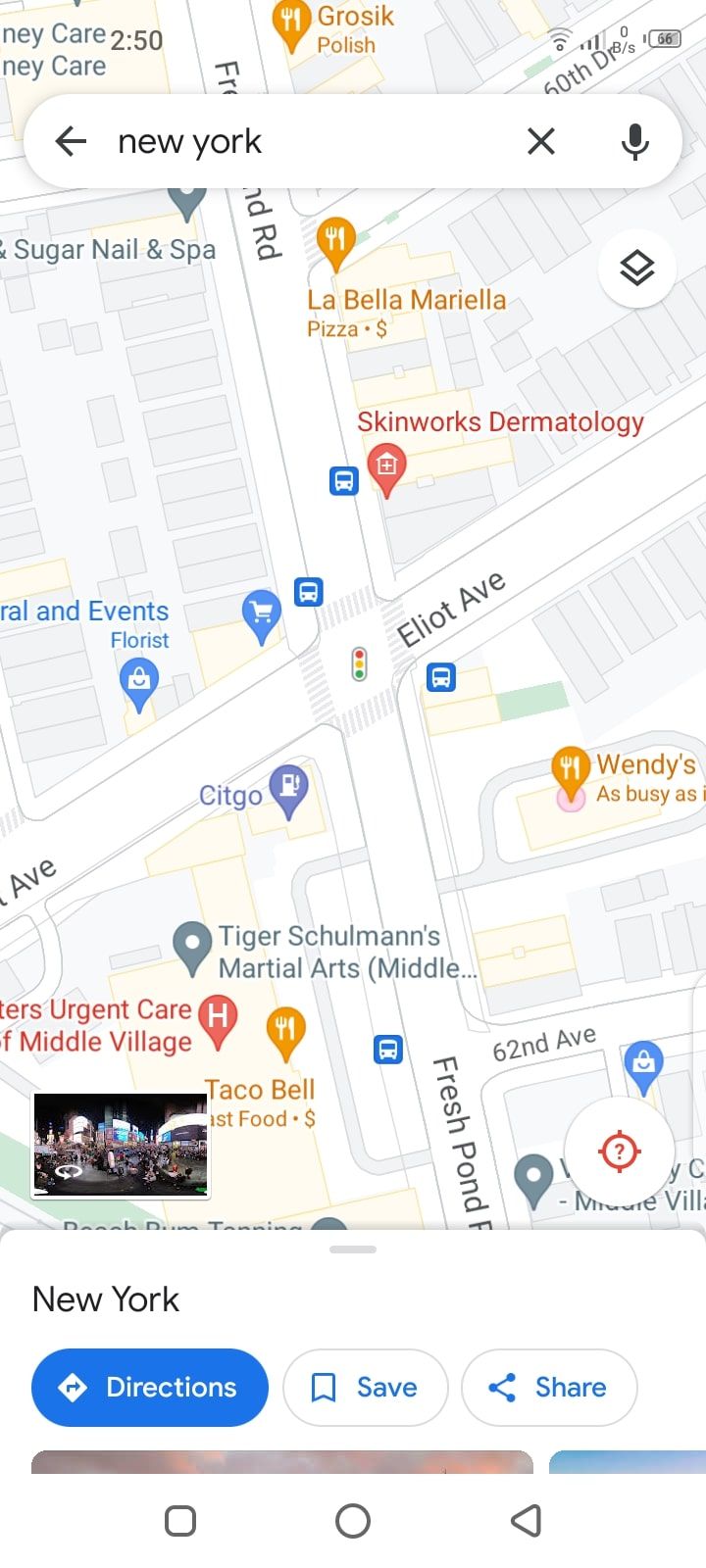This image is a detailed map view of New York City, specifically focusing on a neighborhood that includes landmarks, businesses, and routes. At the top of the picture, the search bar displays "New York" with accompanying navigation options such as a back menu, an X for closing, a microphone icon for voice input, and a search button. Below the search bar, there are options for "Directions," "Save," and "Share."

The map prominently features red and blue lines indicating specific routes, possibly roads or transit lines. Additional navigation icons include a square, a circle, and a back arrow.

Points of interest marked on the map include:
- Groszyk, a Polish food establishment.
- La Bella Mariella, a pizza restaurant.
- Skin Mark Dermatology.
- A visible bus route that runs through Elliott Avenue.
- A nearby florist.
- A Citgo gas station.
- A bustling Wendy's.
- Tiger Schulmann's Martial Arts Middle Village.
- Taco Bell, another fast-food option.

The map also highlights streets such as Fresh Pond Road and 62nd Avenue. A red directional compass shows the cardinal points, allowing for navigation in all directions—north, south, east, and west.